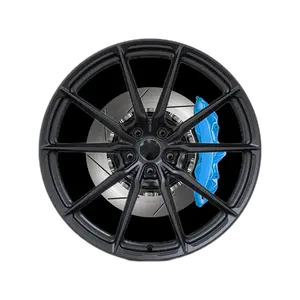This color photograph shows a top-down frontal view of a black wheel rim without an attached tire, set against a white background. The rim is composed of ten distinct black spokes radiating from a hollow center, forming V-shapes around the circumference. Inside the black rim, there's a silver metallic disc brake adorned with diagonal lines, resembling a camera shutter or spiral cuts, creating a detailed flower-like pattern at the center. On the right side of the silver disc brake, a sky-blue component—possibly a brake pad or something decorative—is visible. The silver section also features five evenly spaced holes, presumably for bolts or lug nuts. The entire assembly appears in pristine condition, potentially suitable for a sports car or hot rod, and overall, the image has a somewhat computerized, illustrative appearance.